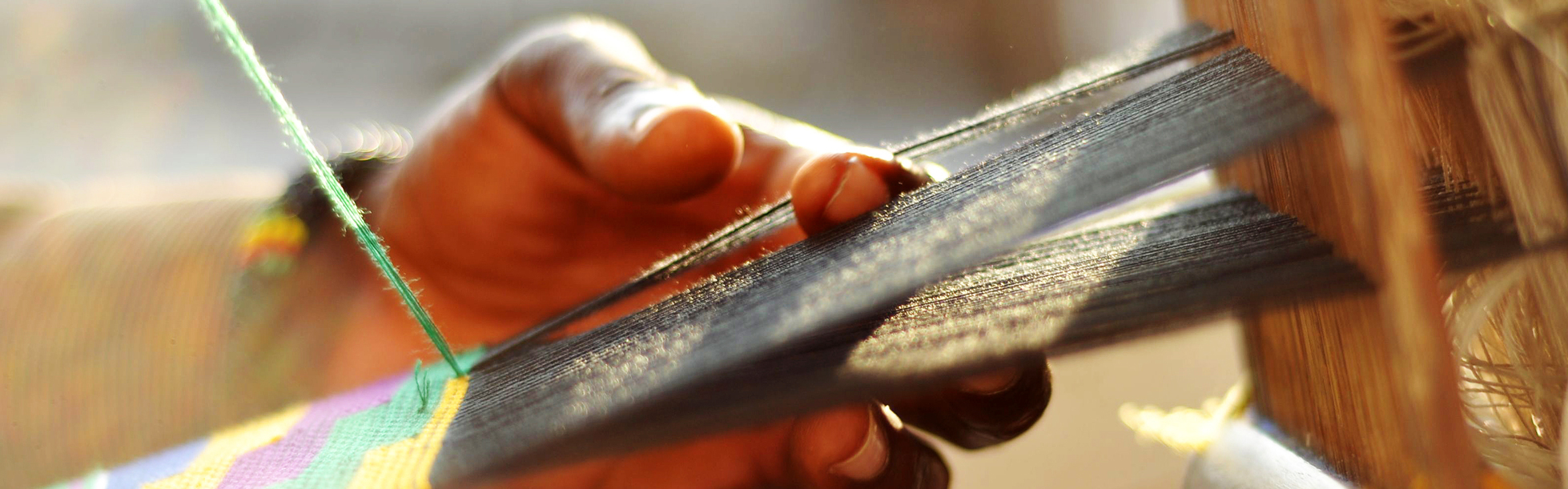In the photograph, a person’s left hand and a portion of their forearm are captured from the left side of the frame, engaged in a precise act of weaving. The hand is manipulating various strings within a wooden weaving loom that occupies the right portion of the image, extending vertically from top to bottom. Two bands of silver yarn are prominently visible, projecting upward from the lower left corner toward the upper right. These yarns are threaded through the loom in a manner that maintains their alignment.

The hand is actively weaving vibrant colored geometric designs into the fabric. These designs, resembling steps, feature an array of colors including light purple, yellow, darker purple, blue, and green. The colored yarn, meticulously integrated into the black string fibers of the loom, progresses from left to right, showcasing a gradient of hues. A green thread also extends upwards, indicating the continual process of manipulation as the weaving progresses. The overall scene captures the intricate artistry and concentration involved in the weaving process.